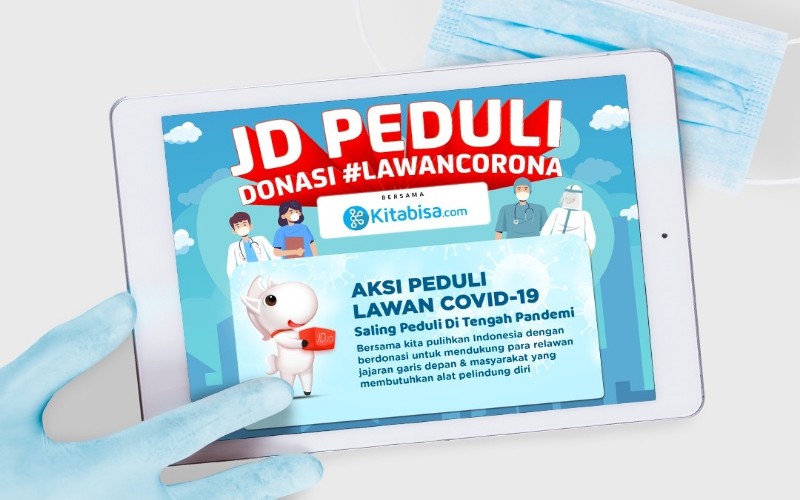The image features a close-up view of a gloved hand positioned in the bottom left corner, distinctly wearing a light blue latex glove. Adjacent to this, occupying the top right corner, is a typical light blue surgical mask with white ear loops, partially covered by the gloved hand. 

Dominating the center of the image is a rectangular, smartphone-like device tilted slightly so that the top is pointed towards the right. The device has a metallic border and rounded corners, highlighted by a light gray background. The display screen prominently features red and white extruded lettering reading, "J.D. Peduli," and additional smaller text below stating, "Donasi Lawan Corona Bersama Kitabisa."

Below this text, there's a white rectangle containing a cartoonish image of a white horse with a black mane, red muzzle, and black hooves, standing upright like a human and holding a red box. This section includes the blue text, "Aksi Peduli Lawan COVID-19," which translates to "Action to Care Against COVID-19."

Surrounding the primary text on the device are small illustrations of medical personnel: a doctor in a white lab coat with a stethoscope, another figure possibly female with a blue smock and mask, and a fully masked medical professional in a white gown with a blue head covering. The detailed scene continues in the background with faint outlines that might represent buildings and cloud formations, contributing to the overall theme of the illustration.

The cumulative elements of the image – the prominent gloved hand, the face mask, and the detailed visual content displayed on the device – suggest it is an informative or promotional piece related to COVID-19 awareness and response efforts in Indonesia, emphasizing community involvement in combating the pandemic.